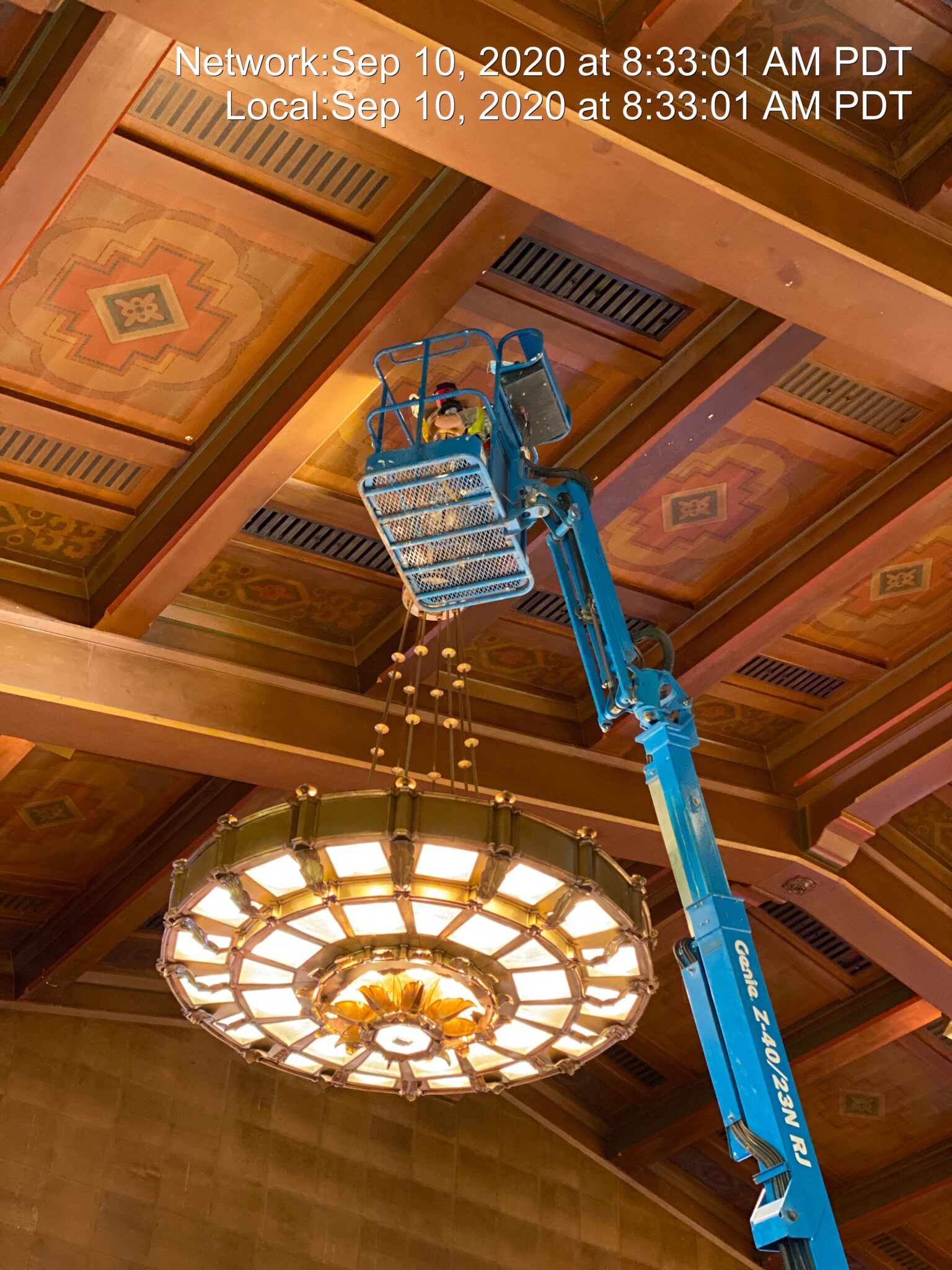The photograph captures the intricate interior of a large hall, possibly a train station or a grand room, emphasizing its expansive and elaborately detailed ceiling. Central to the image is a blue crane, with the model name “Genie Z-40/23NRJ” inscribed in white on its arm, extending from the lower right corner and elevating a worker in a bucket towards the ceiling. The worker appears to be tending to a sizeable, elegant chandelier hanging from the ceiling. This chandelier, which is composed of multiple sections of white glass framed by gold spikes and a surrounding gold circle, showcases a sophisticated design devoid of hanging crystals. 

The ceiling itself is grandiose, featuring patterns within rectangular sections that are likely framed by a metal structure with bronze tinting, mimicking deep wood tones, or possibly actual wood and metal combinations. The ceiling beams are thick, with recessed rectangular panels, and ventilation grates situated along both sides for airflow. Some ducts are visible extending from these sections. The bottom part of the photograph reveals a brownish-tan or gold-toned wall.

The image also includes overlaid white text at the top, with timestamps indicating the photo was taken on September 10, 2020, at 8:33:01 AM PDT.